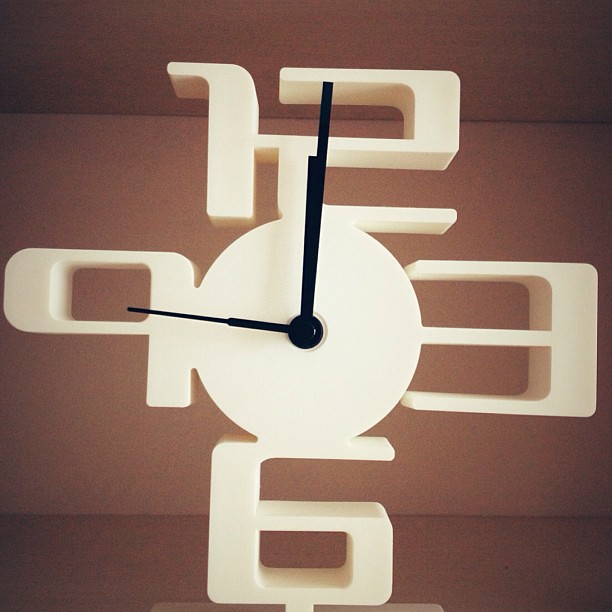This indoor photograph captures a modern, non-traditional clock made from either white-painted wood or plastic, filling the entire frame. Against a light tan, possibly cardboard box background, the slightly grainy and out-of-focus image exhibits the clock’s distinct design. The numbers 12, 3, 6, and 9 are cut out from the white surface of the material, creating a three-dimensional look with soft curves. The clock’s black hands – hour, minute, and second – emerge from a central circle, displaying 12 o'clock with the second hand pointing to the 9, creating a unique and artistic timepiece. There are no other markings or text on the clock, emphasizing its minimalist aesthetic.